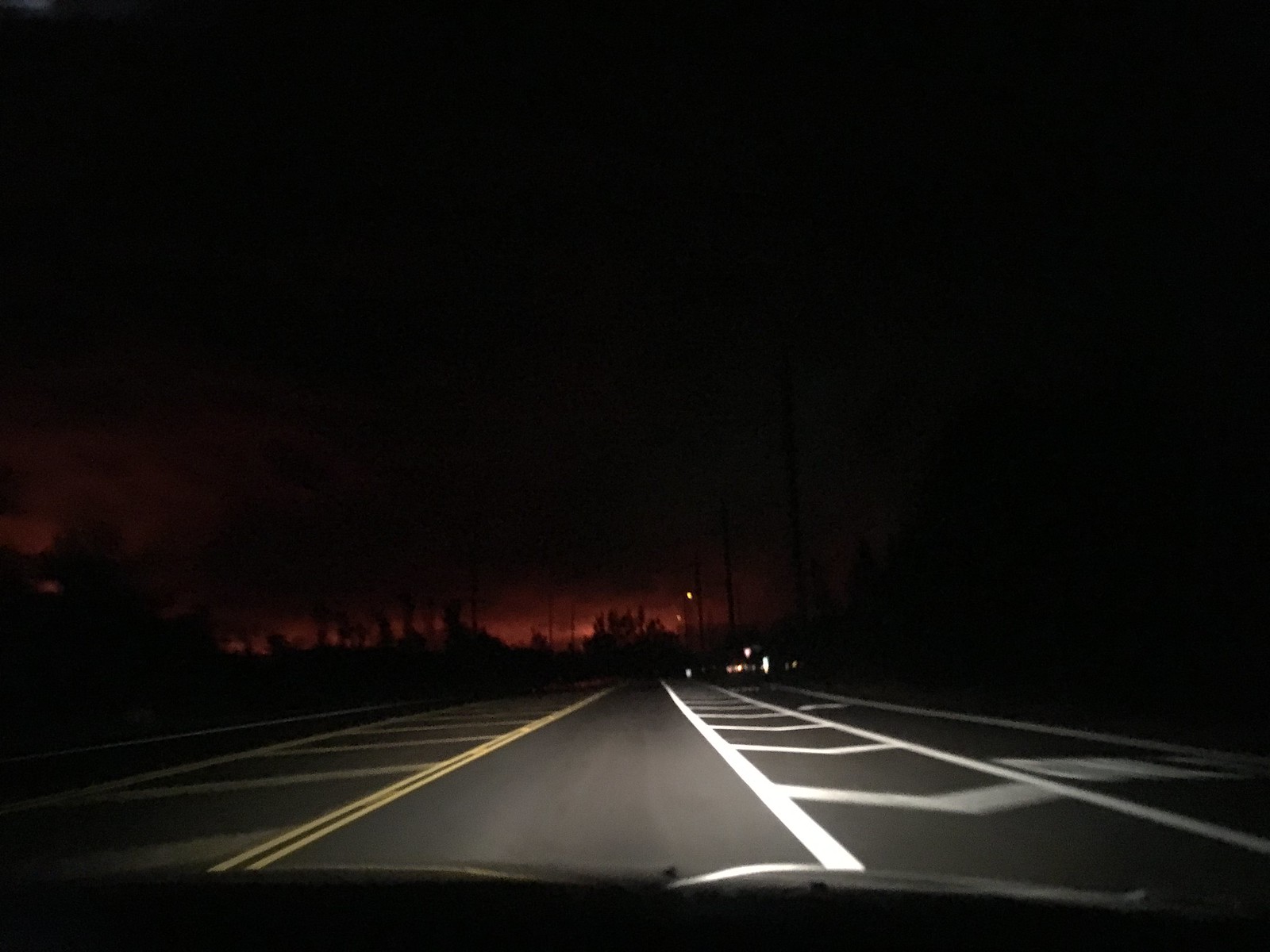This image captures a nighttime scene on the highway from within a vehicle, presumably from the driver's perspective, looking out through the windshield. The well-lit road ahead showcases multiple lanes adorned with both yellow crossing and white lane lines. Despite the night setting, the horizon bursts with dramatic visual contrast as a fiery sunset—its vibrant reds and oranges—dominates the skyline, almost giving the illusion of a distant fire or a city underglow. Silhouetted trees or foliage can be seen against this vivid backdrop. 

Streetlights dot the highway, with most illuminated, casting a glow over the road, although some poles appear unlit. The headlights of the vehicle light up the immediate path ahead, clearly illuminating the chrome windshield wipers and confirming the sharp clarity of the view through the windshield. In the distance, the lights of what seems to be a gas station or a home pierce the darkness. The detailed road markings include a prominent bike lane on the right and a heavily marked section with V-shaped horizontal lines between two vertical lines, in addition to the solid double yellow line indicating no passing. This combination of natural light from the setting sun and artificial light from streetlights and vehicle headlights creates a rich, layered visual narrative of a journey through the deepening night.